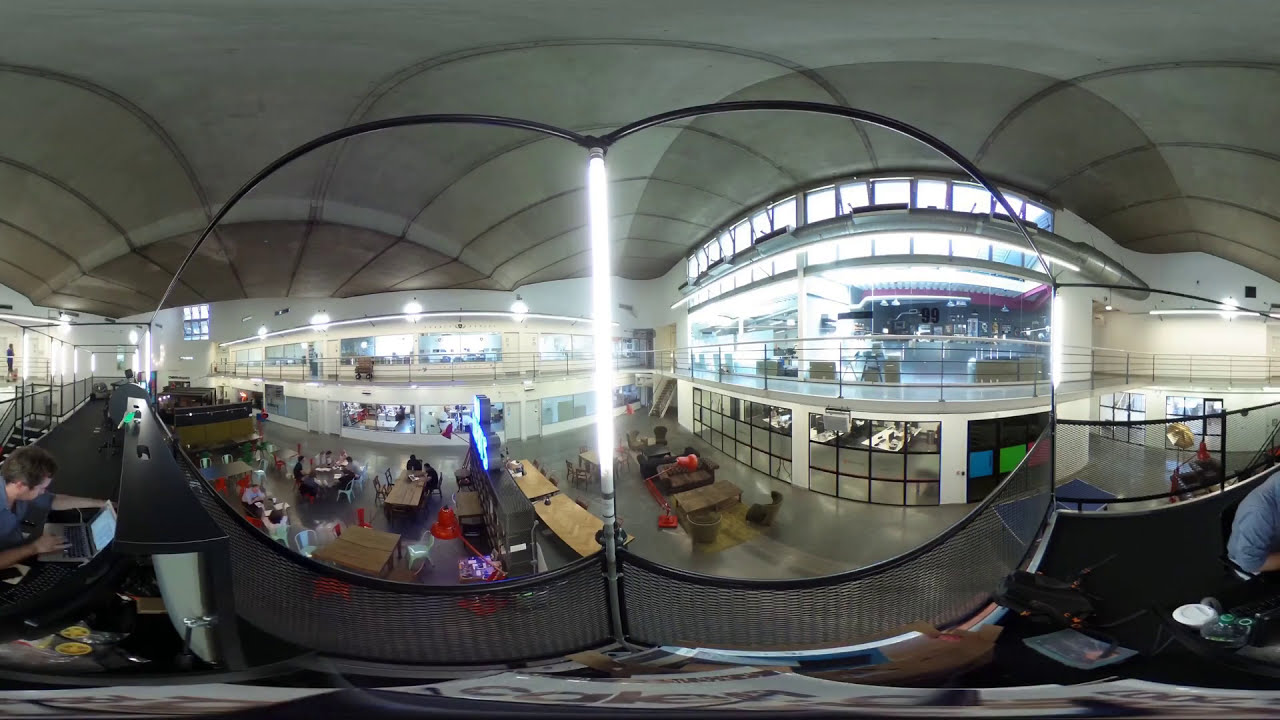The image depicts an indoor scene captured from the second floor of a large, multi-purpose facility that could be a shopping mall, university student union, or community center. The fisheye lens used for this panoramic shot results in significant distortion, making the exact layout and nature of the space somewhat ambiguous. Down below on the first level, several wooden tables are arranged in rows, surrounded by people, many of whom are using laptops, suggesting it might be a study area or communal workspace. There is a noticeable presence of glass-fronted establishments or rooms on both sides of the open central area, adding to the mall-like atmosphere. The second level where the photo is taken features a black metal railing and black flooring, with a visible staircase on the far left leading up to this level. Overhead, fluorescent lighting is seen both on the ceiling and along the walls, enhancing the bright and open feel of the space. Though there's a neon sign visible in the middle, its specifics remain unclear from this angle. Overall, the area is reminiscent of a food court but has a significant focus on study or work activities, potentially indicative of a multi-functional community hub.